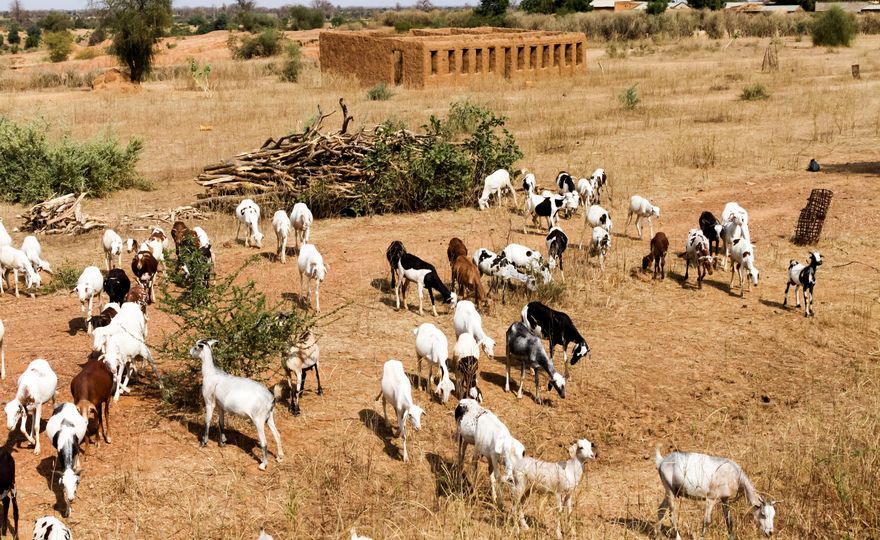The photograph is an almost aerial view of a barren, dusty brown field with a herd of approximately 20 to 50 goats of various colors, including black, white, brown, and mixed patterns, grazing on the sparse grass and thin branches. The rectangular image features occasional tall yellow grasses and spiky bushes scattered around the area. Towards the top center of the frame, there's an old, roofless rectangular building made of tan-colored mud, with multiple window and doorway openings on its sides, reminiscent of an adobe structure. Further back, especially in the top right corner, modern rectangular houses with rusting steel roofs can be seen, along with more trees in the background. In the top left, a larger green spiky tree stands out. The overall landscape appears largely barren and desolate, with no human presence visible.